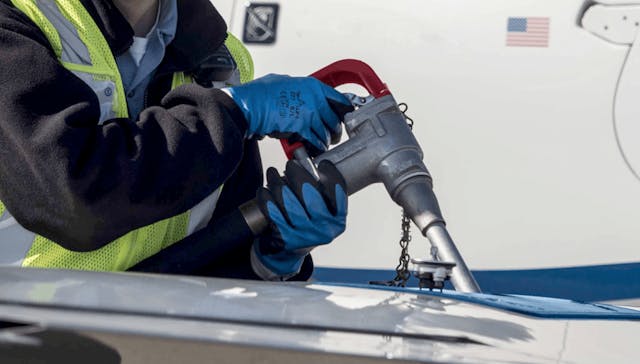In this outdoor daytime photograph, a person, potentially male, is seen refueling what appears to be a white airplane. The individual is standing on the left side of the frame, wearing a distinctive yellow and white mesh safety vest over a black jacket and layered blue and white shirts. They are also wearing blue gloves. The person is holding a fuel pump device with both hands, the right hand pulling a red handle on a silver metal head while the left hand supports the bottom of the pump. The fuel pump is connected to a blue tube that extends out of the frame. 

The airplane being refueled has a small American flag decal and a horizontal blue stripe running along the fuselage, with a visible white wing extending out. Part of the blue metal hatch where the fuel is being pumped into can also be seen. In the background, there are shadows cast by the sun, suggesting a clear day. The scene is set against a backdrop that includes another white vehicle, indicating the location might be an airport or similar facility. No text is visible in the image.